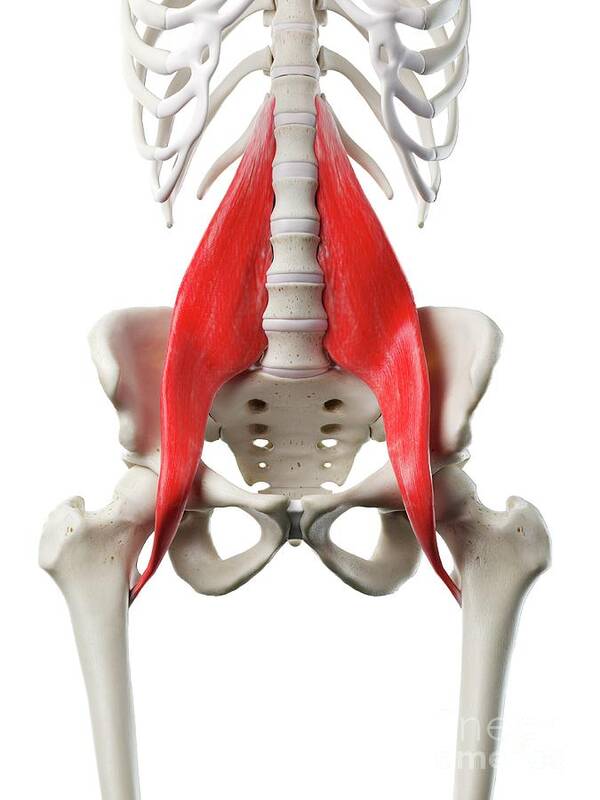This detailed color photograph showcases an anatomical model of a human skeleton, viewed from the mid-ribcage down to just above the kneecaps. The image prominently features the psoas muscles, depicted in a shiny reddish-pink, against the otherwise all-white skeletal structure and plain white background. The psoas muscles are shown originating from the lumbar spine, coursing through the hip girdle, passing the pelvis, and terminating near the top of the femurs on either side. The rest of the skeleton, including the ribcage, spine, pelvis, and femur bones, is rendered in white, making the highlighted psoas muscles the focal point of the image. There are no additional features, text, or background details present, emphasizing the anatomical connection from the spine to the femurs.